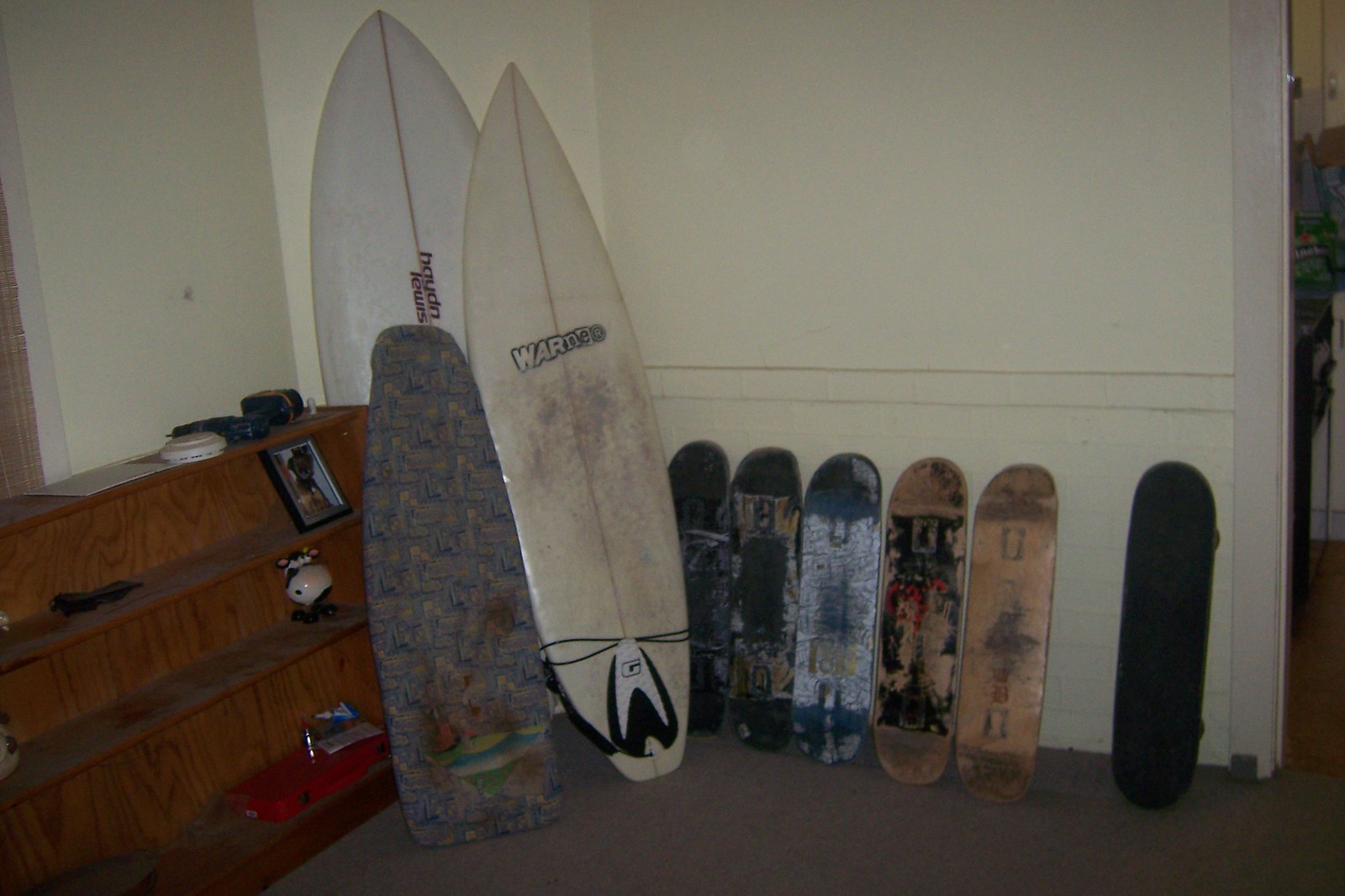In this photograph, taken indoors in a somewhat dimly lit room, several items are leaning against the walls, creating a scene of organized clutter. The background is a beige or off-white wall, adorned with some paneling in the middle, and the floor appears to be brown.

On the right side of the image, six skateboards are lined up, leaning against the wall. They vary in appearance, with one skateboard distinctly black and others showing signs of wear with multicolored textures. Adjacent to the skateboards, two large surfboards, also worn out and off-white though of slightly different shades, stand against the corner of the walls.

Towards the left, against the adjacent wall, is a portable ironing board with a ripped cover that features a blue and red pattern, as well as signs of burn marks. The ironing board leans against a brown wooden dresser with two shelves and a bottom compartment. The top shelf holds a framed photo and a round ceramic decoration, while the lower shelf contains a red box. Atop the entire scene, a smoke detector is visible on the ceiling, hinting at the indoor setting.

This image captures an eclectic collection of skateboards and surfboards, accompanied by an ironing board and a cluttered wooden dresser, against a backdrop of beige walls and a brown floor.